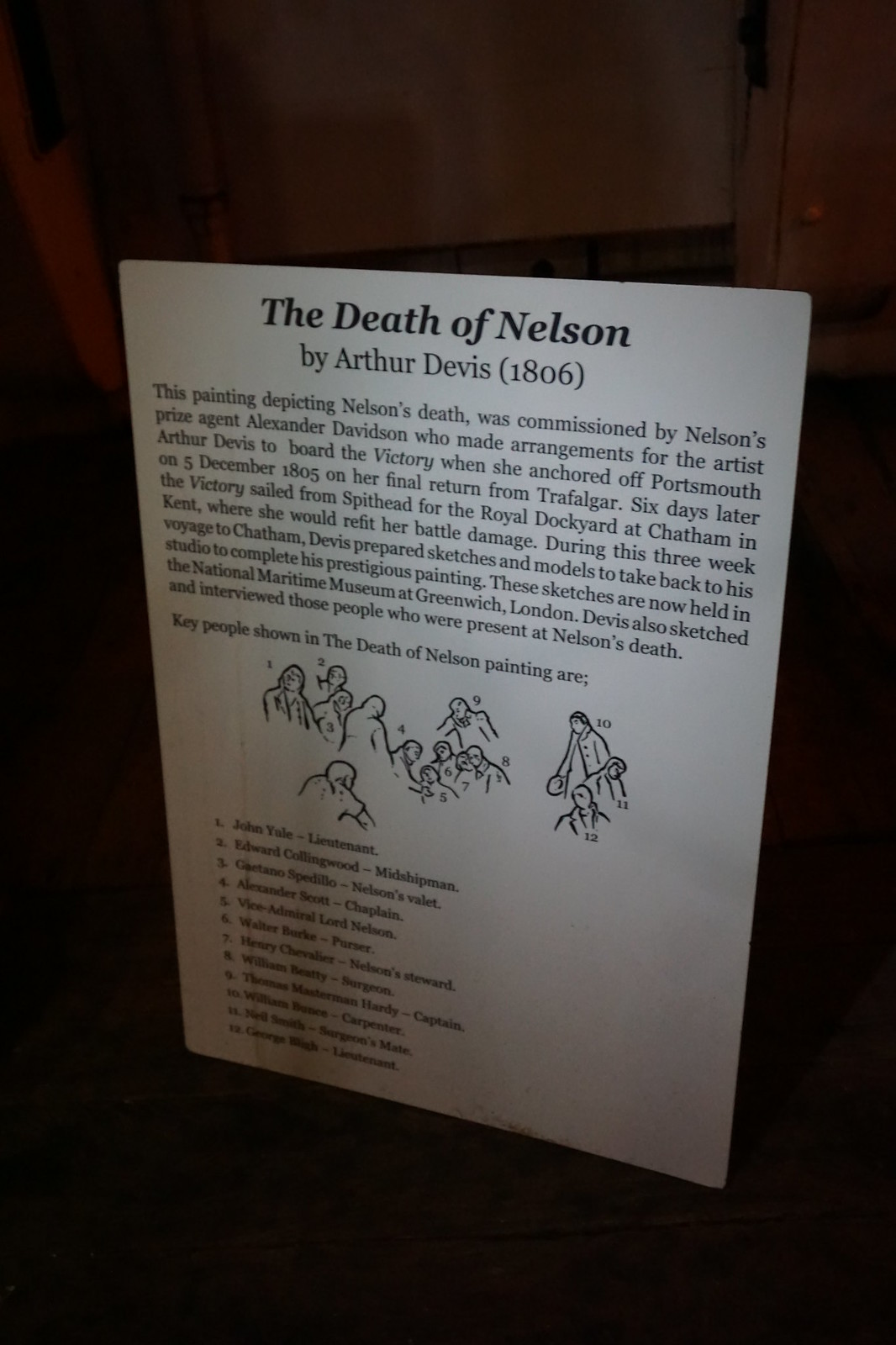A detailed descriptive caption for the image based on the combined information would be:

"This image features a piece of paper prominently displayed on what appears to be a window, possibly in an art gallery or museum setting. The paper, illuminated against a contrasting dark background, bears the title 'The Death of Nelson by Arthur Davis, 1806.' The document explains that the painting, depicting the death of Admiral Nelson, was commissioned by Nelson's prize agent, Alexander Davison. Arrangements were made for artist Arthur Davis to board the HMS Victory when it anchored at Portsmouth on December 5, 1805, following its return from the Battle of Trafalgar. After six days, the Victory sailed from Spithead to the Royal Dockyard in Chatham, Kent, for repairs. During this three-week voyage, Davis created sketches and models, which he would later use in his studio to complete the prestigious painting. These preparatory sketches are now housed at the National Maritime Museum in Greenwich, London. Davis also conducted interviews and produced sketches of several individuals who were present at Nelson's death scene. Additionally, the lower section of the paper lists key people depicted in the painting. The background details are sparse due to the dark setting, but a white or tan door with a handle is visible behind the paper."

This caption integrates the primary details emphasized in both verbal descriptions, combining them into a coherent and thorough account of the image’s content and context.